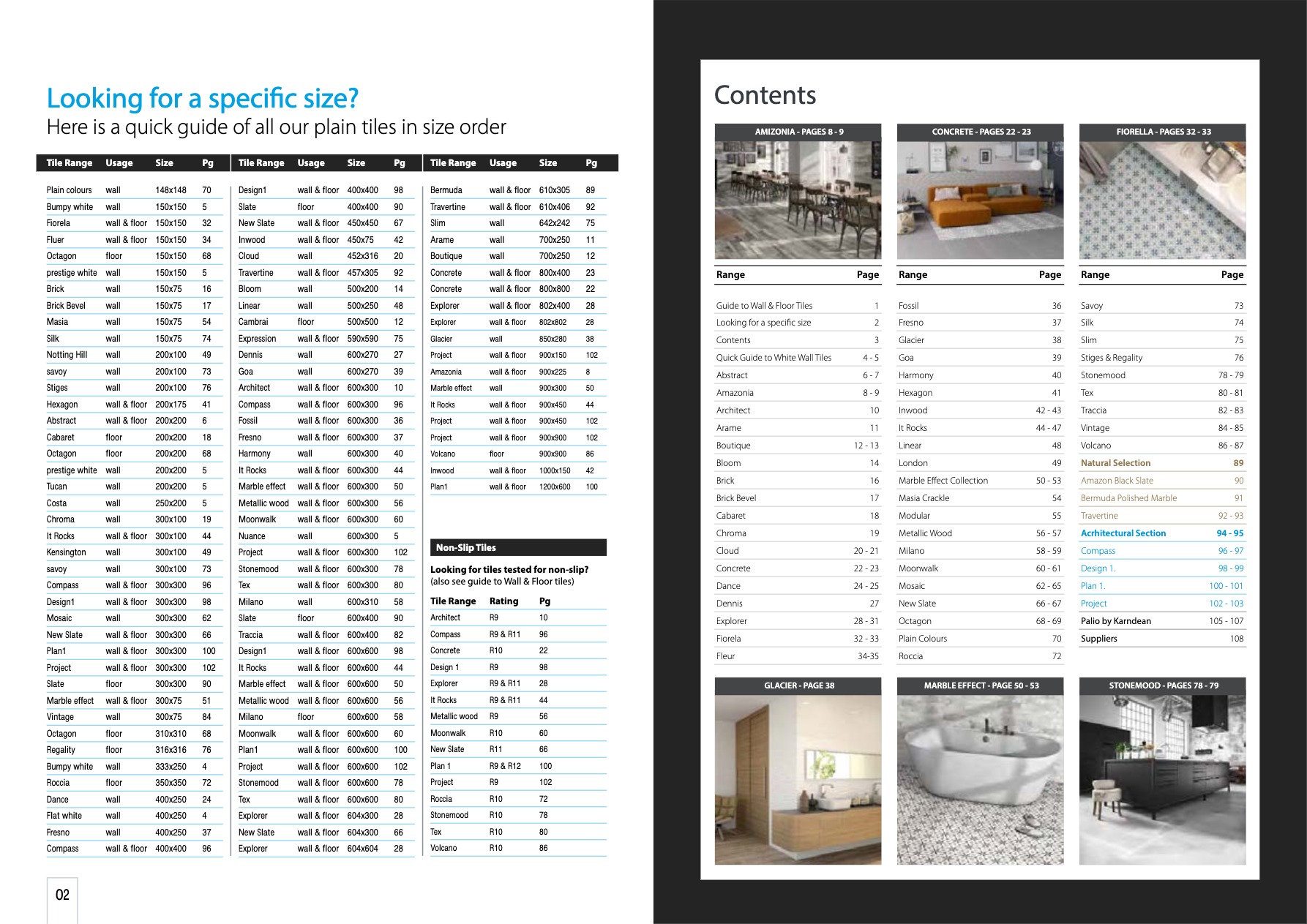The provided image features a detailed guide for selecting tiles. On the left side, there's a section titled "Looking for a specific size? Here is a quick guide to all of our plain tiles in size order." This section organizes tiles by range, usage (wall or floor), and size, with three columns of tiles listed. Additionally, non-slip tiles are separately categorized with their ratings. This comprehensive list includes approximately 60 different tiles.

On the right side, there's a "Contents" section featuring images of various tile styles named "Amazonia," "Concrete," and "Marilla," all of which are suitable for flooring. Each style is accompanied by a page range, indicating where detailed information about these tiles can be found. Below this section, there are visual examples showcasing how these tiles can be used in different settings, providing inspiration and guidance for potential buyers.

Overall, this image serves as a thorough resource for anyone looking to purchase tiles, particularly for flooring, offering a wide variety of options and practical guidance.